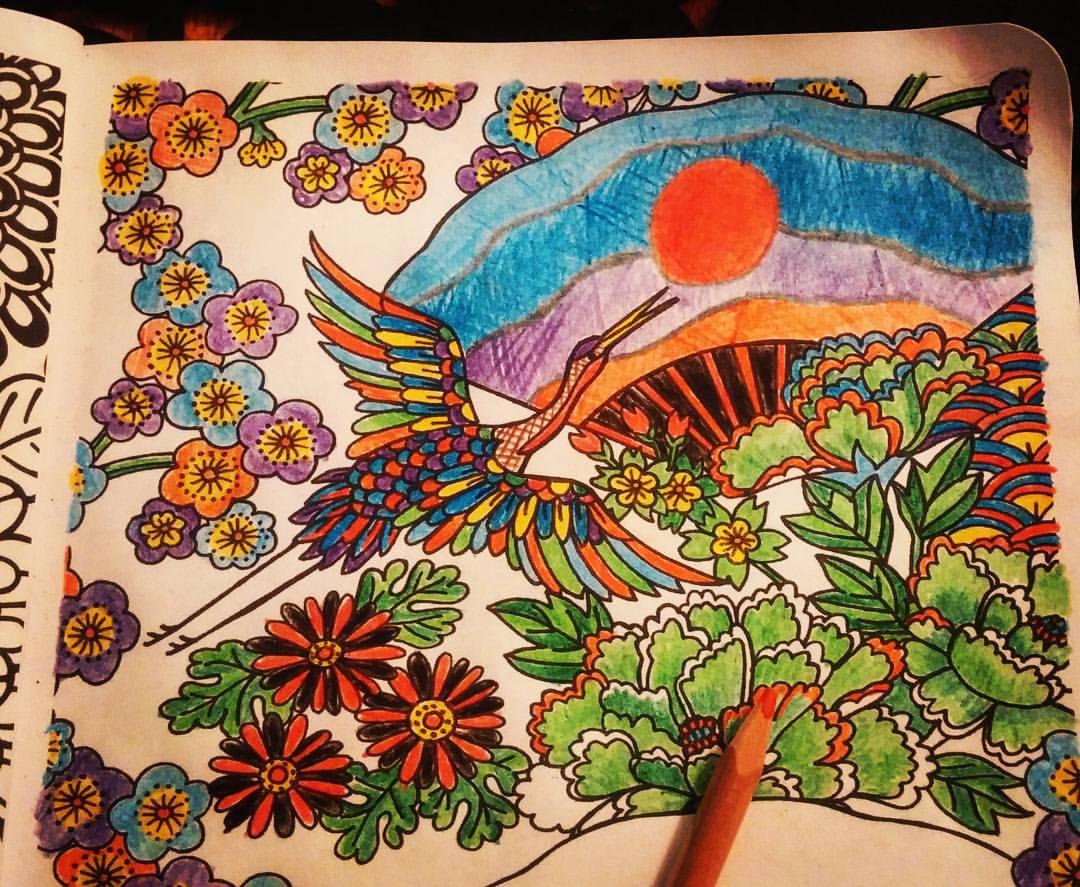The image appears to be a vibrant, mixed-media drawing created with crayons, colored pencils, and possibly paint, possessing an intricate blend of textures and styles. Dominating the scene is a crane, rendered in an array of vivid hues—reds, blues, greens, yellows, oranges, and purples—soaring upward with its wings majestically spread. The crane evokes the mythical imagery of a phoenix, highlighting its significance amidst a landscape teeming with life.

Beneath the crane, the landscape flourishes with an abundance of colorful flowers and a verdant forest, painted in an array of greens, purples, yellows, reds, blues, and blacks. Rising through this sea of flora is a detailed, handheld fan—distinctively outlined with wooden patterns. The fan showcases an intricate design that stretches across multiple layers: the top layer depicts a bright, red-orange sun glowing in an expansive blue and orange horizon, while below it, a deep purple mountain range adds a sense of depth to the composition.

This artwork, possibly originally a page from a coloring book that has been meticulously filled in, presents a theme of nature and mythical beauty, harmoniously interwoven. An orange pencil lies atop the drawing, hinting at the creative process, adding an authentic touch to the final, untouched sections of the page which contrast with the vibrantly filled areas. This detailed scene captures a moment of intense color and vitality, encapsulating an imaginative interplay of natural and mythical elements.